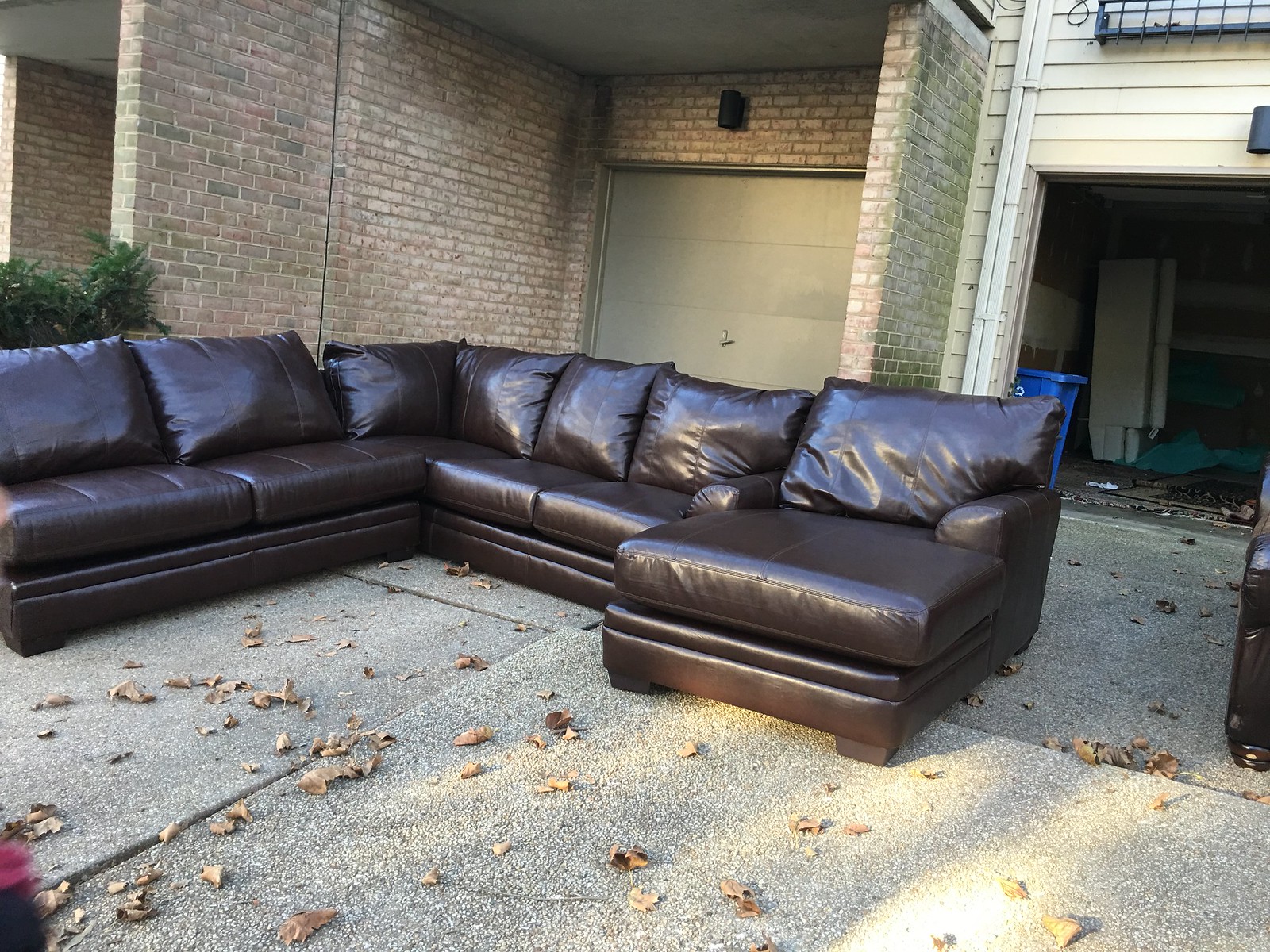A peculiar photograph captures a large sectional couch positioned outside in a driveway, in front of a light-colored brick building with evident features that hint at a residential setting. The sectional couch, crafted in dark brown pleather, glistens under the light, emphasizing its shiny texture. The couch is arranged in an offset U shape, comprising three sections: the left section has two cushions and two headrests; the middle section consists of three cushions with three headrests, while the right section extends with one cushion, one headrest, and a footrest.

The driveway, constructed from grey concrete, displays signs of wear with uneven cement and scattered brown leaves, suggesting a fall setting. In the background, a two-car garage with one door open reveals a green tarp on the floor and a blue recycle bin to the left of the open door, while the closed door remains adjacent. Above and around the garage, the light yellow siding contrasts slightly with the light brown brick construction, enhancing the detailed context of the scene.